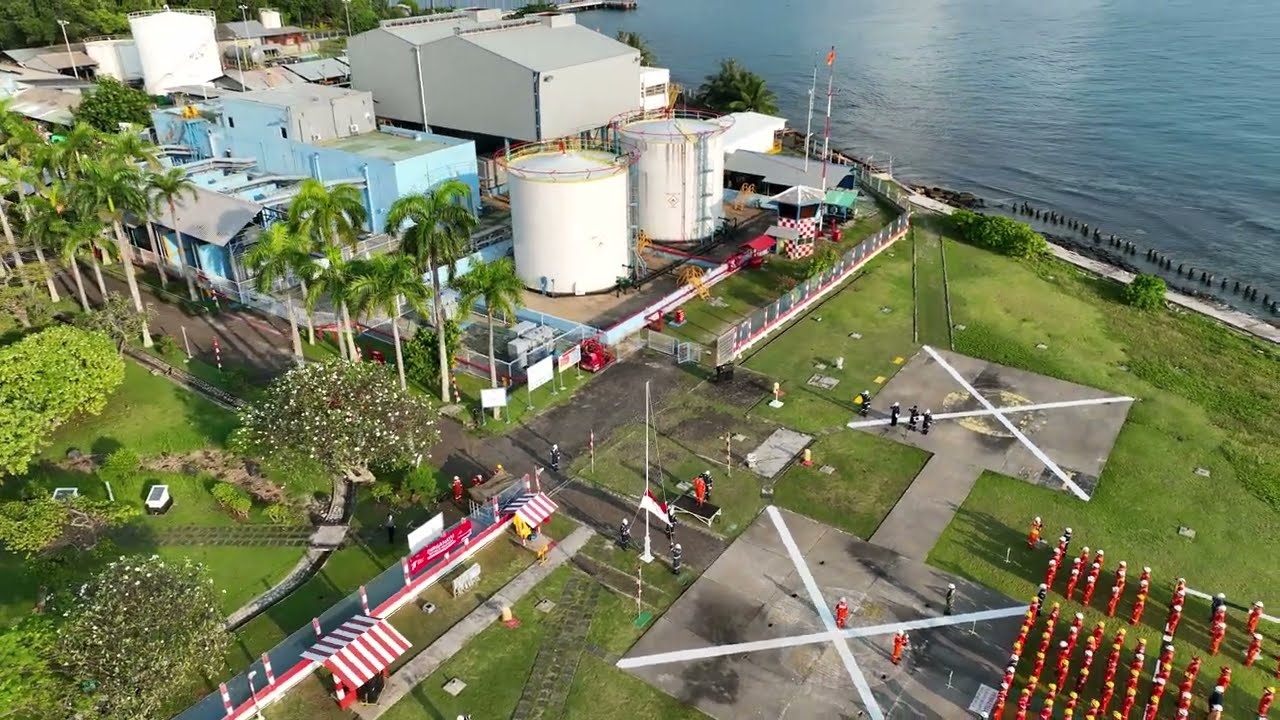The image presents an aerial view of a coastal industrial plant situated in a likely tropical climate. The scene is divided into several distinct areas: at the top left, a cluster of industrial buildings painted white and light blue is prominent. Below this industrial zone, stretches of green grass and clusters of trees and bushes, including palm trees with brown trunks and green tops, add a natural contrast. To the top right, a body of blue-green water extends outward, and at the bottom of the water, brown logs or similar objects are partially submerged.

Adjacent to the water, a gray sidewalk and a black or gray pathway weave through the scene, flanked by various patches of green foliage, including a distinct field and isolated bushes. There’s a cement area resembling a dumbbell shape with white X markings, populated by people in black and red clothing, likely indicating a band or team in preparation for an event. Nearby, red and white canopies dot the grassy sections, providing shade for the individuals.

Additional structures include white water towers in the industrial area and another red and white checkered canopy tower. More trees and grassy areas frame the left side of the image, enhancing the tropical ambiance. The overall scene lacks any textual elements, allowing the blend of natural and industrial features, as well as the human activity, to stand out vividly.